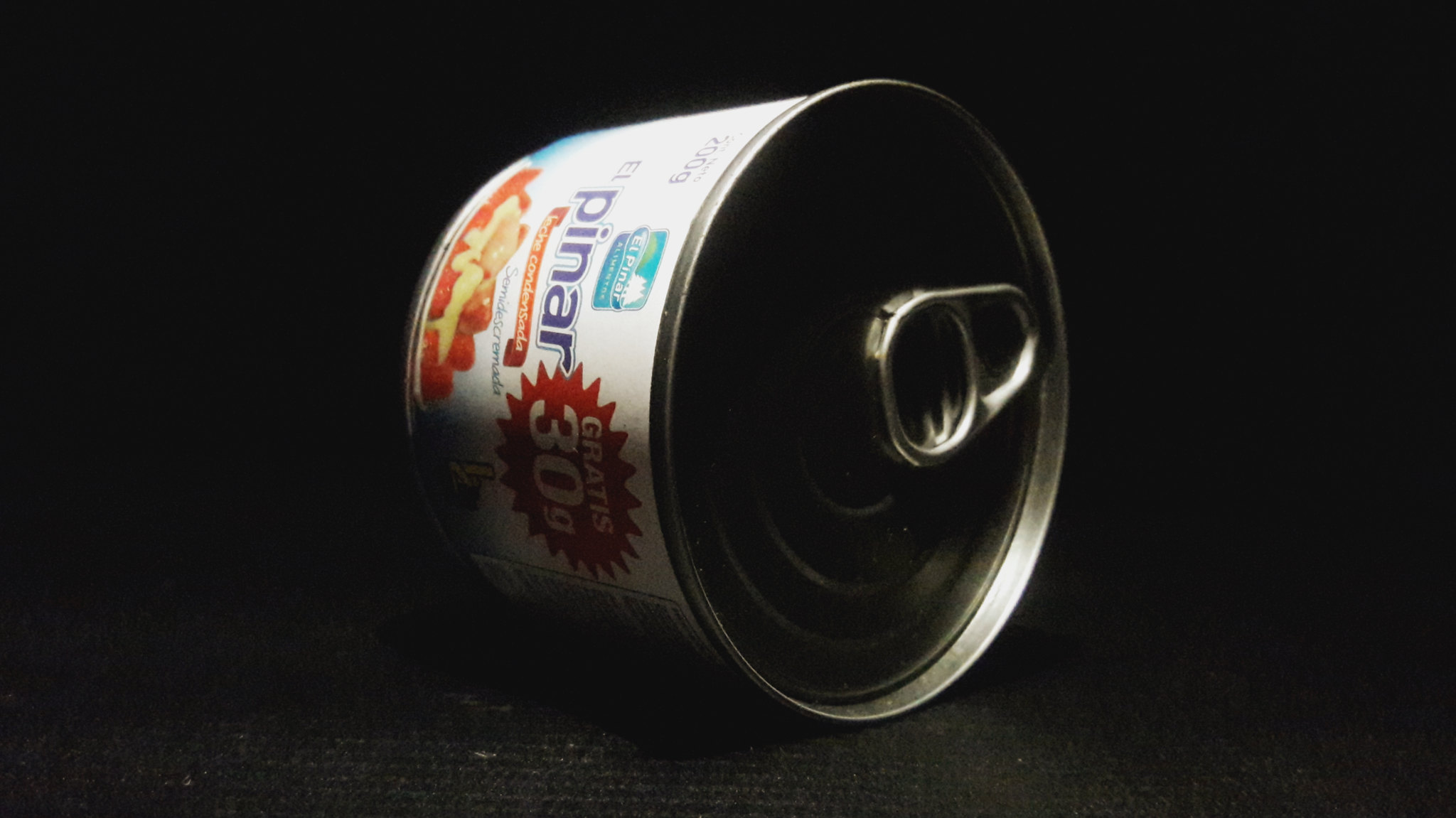The photograph, taken indoors with professional lighting shining from the top left, features a can of table cream or sweetened condensed milk resting on its side. The can, identified as El Pinar, is silver with a pull tab for easy opening and measures 200 grams with an additional 30 grams gratis. The dark black background and the black textured surface on which the can rests create a dramatic contrast, accentuated by the light, which strongly illuminates parts of the can's label, leading to some areas being bleached out. The label, predominantly in Spanish, showcases an image of strawberries topped with cream, suggesting its usage in desserts. The red and white sections of the label explain that this is a type of concentrated milk, noted for its sweetness, and is typical in dessert recipes.